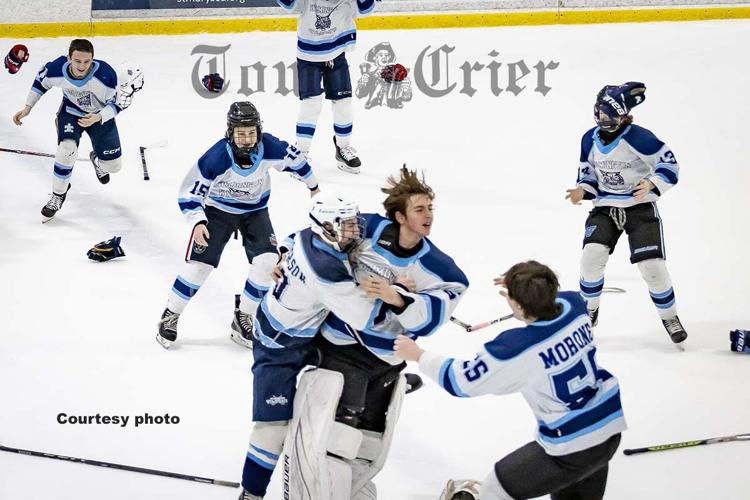This photograph captures a jubilant moment of a hockey team celebrating a victory, likely after scoring a winning goal. The scene is set against a backdrop featuring a watermark with the text "Town Crier," alongside an image of a colonial-era town crier and the words "Courtesy Photo" at the bottom left. The ice is scattered with gear—helmets, gloves, and sticks—abandoned in the frenzy of celebration. 

At the center of the image, the apparent scorer of the winning goal, unmasked and ecstatic, is engulfed in a hug by one teammate, while another skates in to join the embrace. Surrounding them, other players, all wearing white jerseys with blue details, black shorts, and white leg pads accented with blue and black stripes, converge toward the center. One player at the top left is captured in action, tossing his gear onto the ice. Another player to the right celebrates with arms outstretched in amazement. The scene is alive with movement and adrenaline as seven players in total are visible, with one partially obscured by the edge of the photograph.